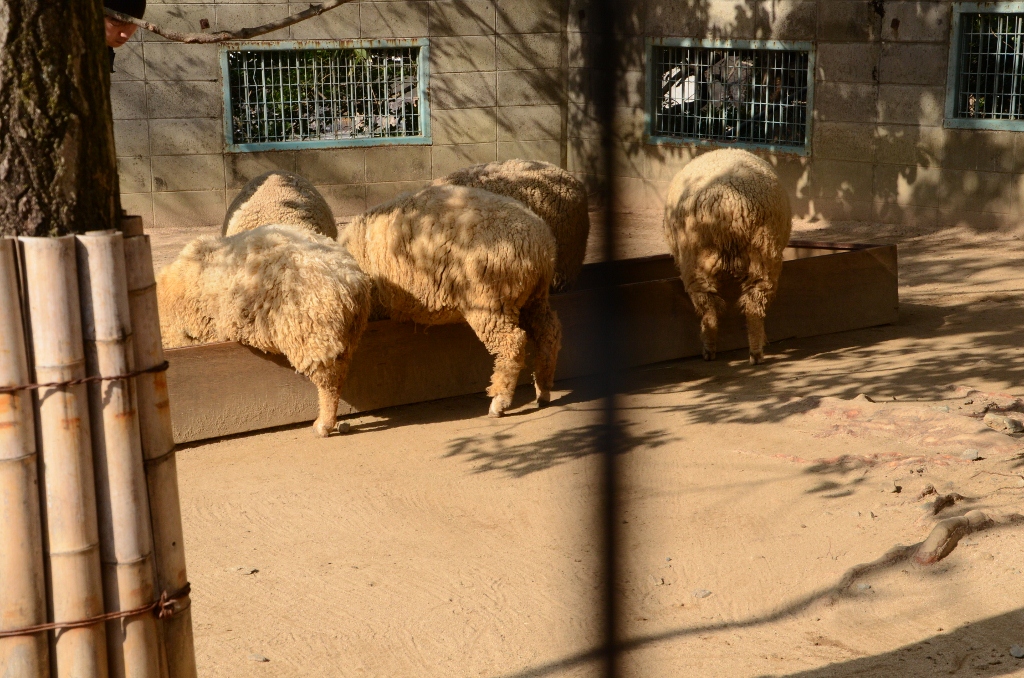The photograph captures a farm or zoo scene with five fluffy, white sheep gathered around a large, brown wooden feeding pen. All the sheep, identifiable by their long wool and tan shades with cream highlights, have their heads lowered, fully immersed in feeding, making only their hind legs and backs visible. The feeding pen is positioned next to a gray cinder block structure with rusted, green-barred windows. The ground surrounding the pen is sandy and devoid of other plant life, except for a single tree on the left side of the frame. The tree is protected by bamboo poles tied around its base, likely to safeguard it from the animals. Shadows on the ground indicate that the photo was taken in bright sunlight. One notable detail is what appears to be a black line in the middle of the image, possibly indicating the presence of a fence or an obstruction partially blocking the camera's view.